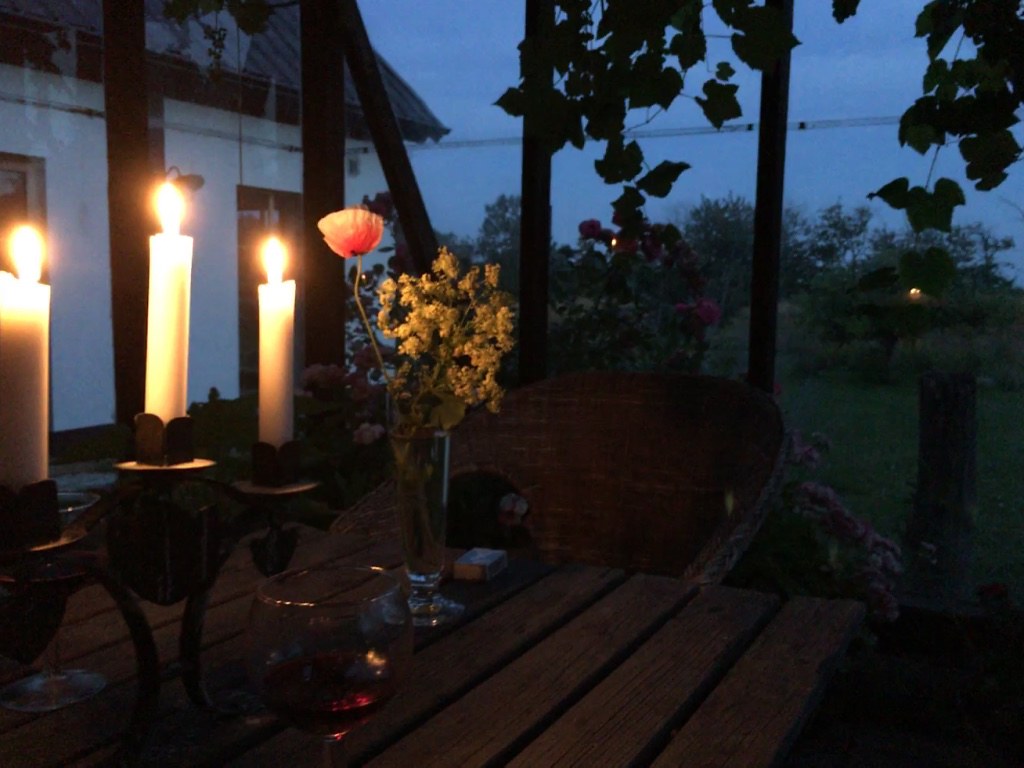The outdoor evening scene captures a cozy and tranquil setting on a wooden deck. A single wicker chair accompanies a wooden slatted table adorned with three lit white pillar candles arranged on a candlestick. The table also holds a half-filled wine glass of red wine and a glass vase containing a single pink flower, possibly a tulip or daisy, surrounded by small white flowers and some greenery. The backdrop reveals the side of a white house with a black roof, partially obscured by a canopy-like structure with wooden posts and hanging leaves. The surroundings include a lawn with scattered flowers, a tree stump near the chair, distant trees, and a visible power line cutting through the evening sky, which deepens to a darker blue, hinting at the approaching night.